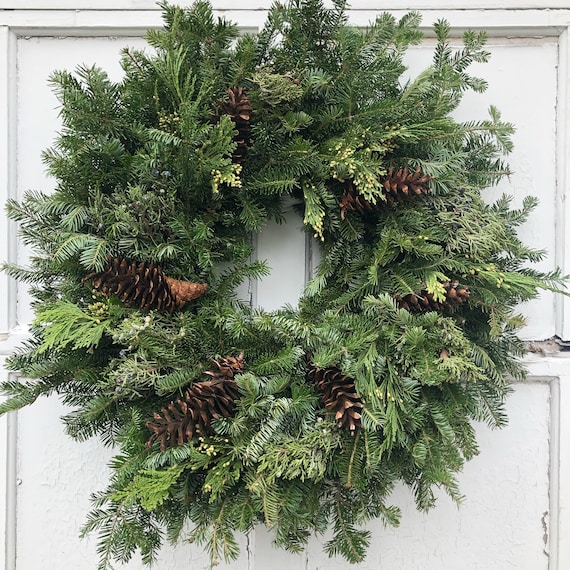This color photograph captures a large, circular, holiday wreath prominently displayed on a white, wooden door. The vivid greenery of the wreath is formed from fresh evergreen leaves and pine needles, giving it a lively and organic appearance. Interspaced among the foliage are several dark brown pine cones, one of which is partially closed, enhancing the wreath's natural texture. The wreath's design features a donut shape with an empty center, seamlessly integrating various types of greenery and ferns. The white door, adorned with square panels, forms a contrasting backdrop that accentuates the vibrant green of the wreath. The overall composition fills most of the frame, portraying the wreath in a realistic and detailed manner appropriate for the holiday season, though it lacks any additional decorations like lights. The photograph is square in format and employs a style of representational realism, convincingly capturing the essence and detail of the festive wreath.